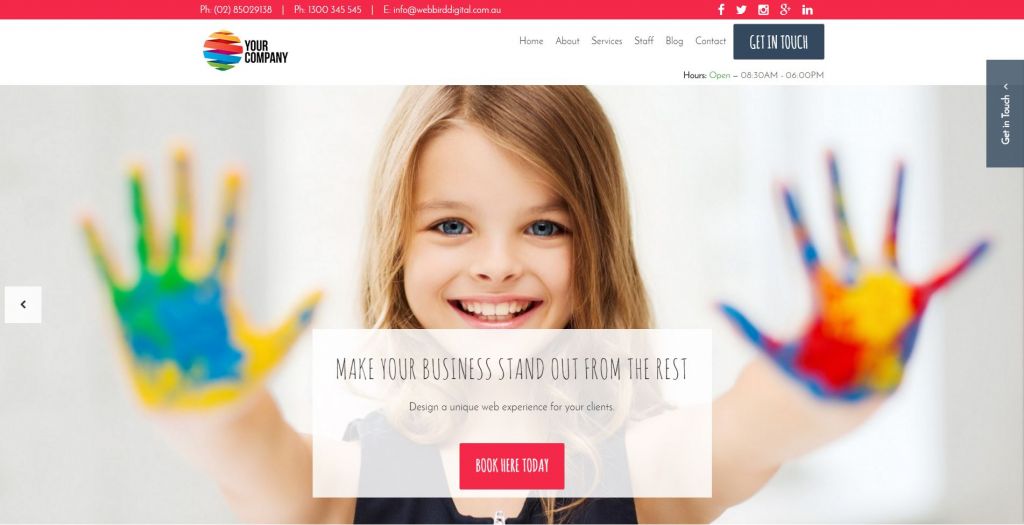Above the top, the image features contact information including phone numbers (0285029138 and 1300-345-045-8), a website link (www.webradigital.com.au), and icons for social media platforms (Facebook, Twitter, Instagram, G+, LinkedIn). The centerpiece of the image is a colorful sphere segmented into orange, red, blue, and green sections labeled with navigation prompts such as "Your Company," "Home," "Services," "Staff," "Blog," and "Contact." Capsulated below this sphere is a section labeled "Get in Touch" with operational hours listed from 8:30 AM to 6:00 PM.

To the right, there is a vertical sidebar once again labeled "Get in Touch." Adjacent to this sidebar on the right, an image depicts a cheerful young girl with short brown hair, prominent teeth, and blue eyes. She is joyfully smiling, and her hands are brightly painted with different colors: her left hand showcases green, blue, and yellow, while her right hand displays colors arranged in blue, red, yellow, and black patterns, forming a fist.

At the center of the image, a text overlay reads, "Make your business stand out from the rest. Design a unique web presence for your clients." A red square positioned below the text prompts, "Book Today." The entire background of the image is colored white, and includes slightly blurry visuals on both the left and right sides, further emphasizing the central elements and text.